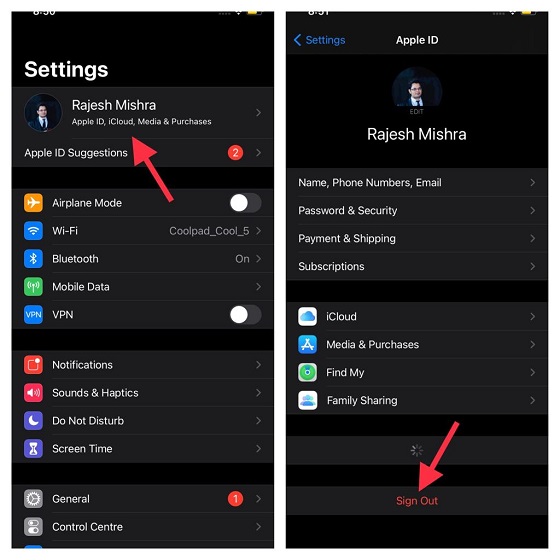This is a dual image presentation, depicting screenshots presumably taken from a mobile phone's settings interface. 

The left image displays the main settings screen, evidenced by a black banner at the top. Below the banner, there is a profile section featuring a user's profile picture—cropped into a circle—and their name, "Rajesh Mishra." Beneath the name, the label reads "Apple ID, iCloud, Media, and Purchases." To the right of the profile section, an arrow icon points right, indicating that it is a clickable area.

Highlighted in this image is a red arrow pointing upwards specifically to the "iCloud" section, suggesting its importance or relevance. The left-hand side of the screen lists various settings options such as "Airplane Mode"—which, like the "VPN" setting below it, shows an off-position toggle button—"Wi-Fi," "Bluetooth," "Mobile Data," "Notifications," "Sounds & Haptics," "Do Not Disturb," "Screen Time," "General," and "Control Center." Notably, the "General" setting is marked with a red notification badge, displaying the number one.

The right image provides more detailed account information. It again features the user's profile image and name, "Rajesh Mishra," followed by sections including personal information (name, phone numbers, email), "Password & Security," "Payment & Shipping," "Subscriptions," as well as app-specific settings like "iCloud," "Media & Purchases," "Find My," and "Family Sharing." A prominent red arrow points down towards the "Sign Out" option, indicating user action.

Together, these images illustrate the settings interface with an emphasis on profile and account management features.